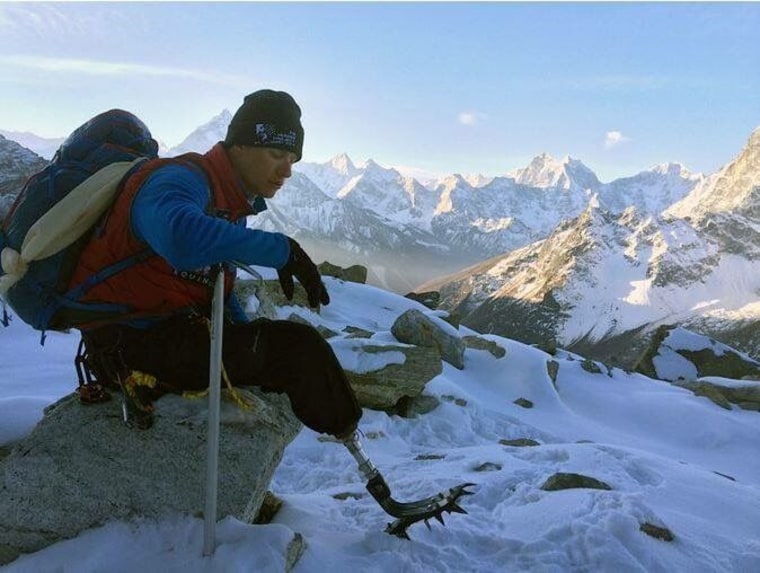In this photorealistic image, a man sits alone on a snow-covered rock high in a vast, snowy mountain range. He is an amputee with a prosthetic leg designed for traction, featuring spikes to navigate the icy terrain. Dressed warmly for the harsh conditions, he wears a black beanie, a red vest over a blue thermal shirt, black gloves, and black pants. The man also carries a blue backpack and leans on a hiking stick, with additional climbing gear, including chains and ropes, attached to his pants. The sky above is clear with a light blue to light purple hue, sporadically dotted with a few clouds. The surrounding landscape is a dramatic expanse of snow-capped, rocky mountains, presenting a serene but formidable backdrop. The man's gaze is fixed on his prosthetic leg, embodying a moment of reflection and solitude amid the majestic wilderness.